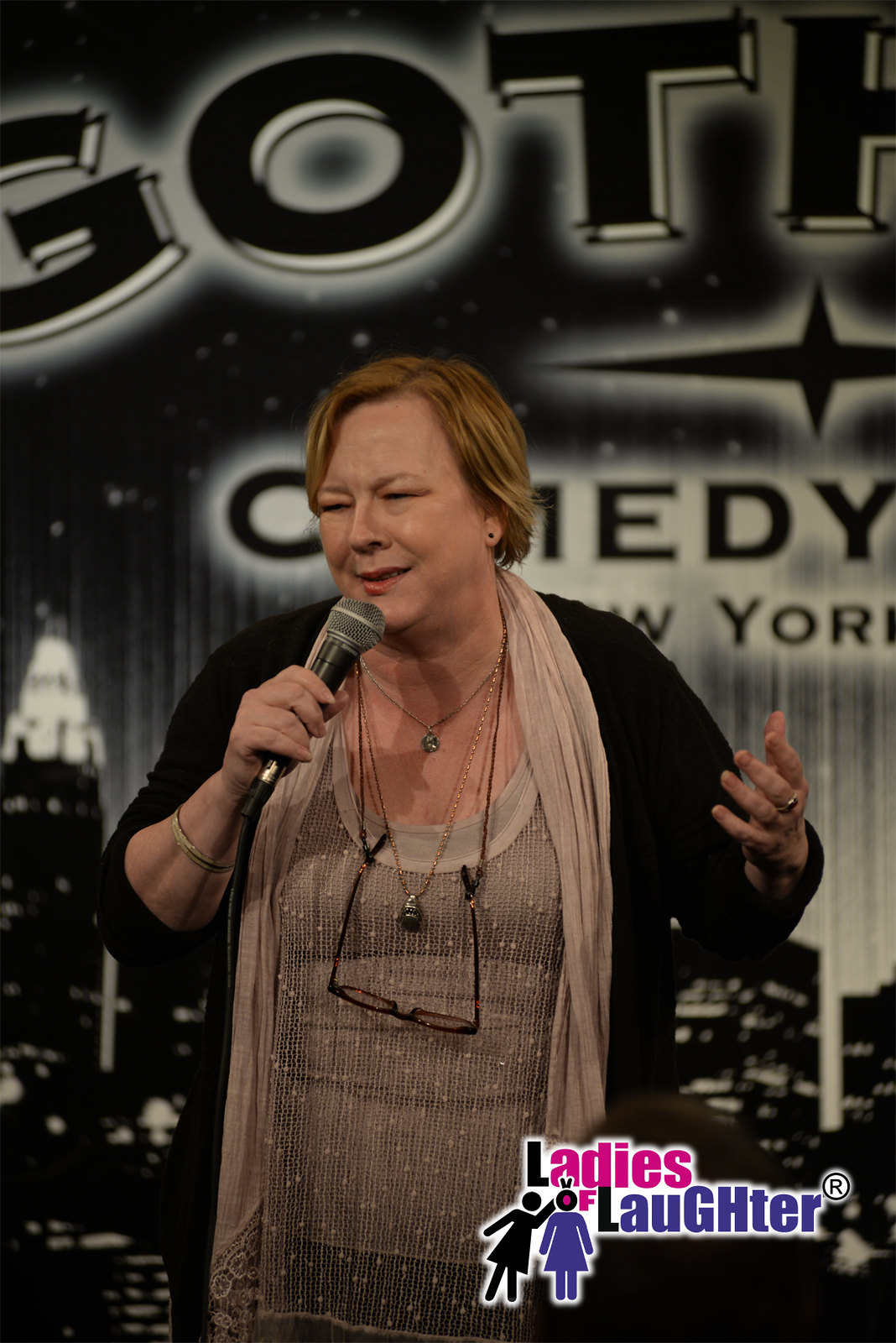In this image, an older woman comedian, resembling a typical, mom-like figure, is performing on stage during the "Ladies of Laughter" comedy hour. She has medium-length hair that is a blend of blonde, reddish, and brown tones. Her white skin is accented with a hint of lipstick. She is wearing a multi-layered outfit consisting of a gray tank top, a knit top, and a black shawl or sweater. Around her neck, she has glasses hanging from a string and a couple of necklaces. The comedian holds a microphone in her right hand, gesturing with her left hand, and her squinted eyes give her an annoyed or expressive look, while her slightly open mouth suggests she is mid-sentence. Behind her, the stage backdrop features a night sky with stars and a cityscape with illuminated skyscrapers, and partially visible text reading "GOT" and "New York" with the word "comedy" beneath. The bottom of the image carries the "Ladies of Laughter" logo, along with small images of two women.